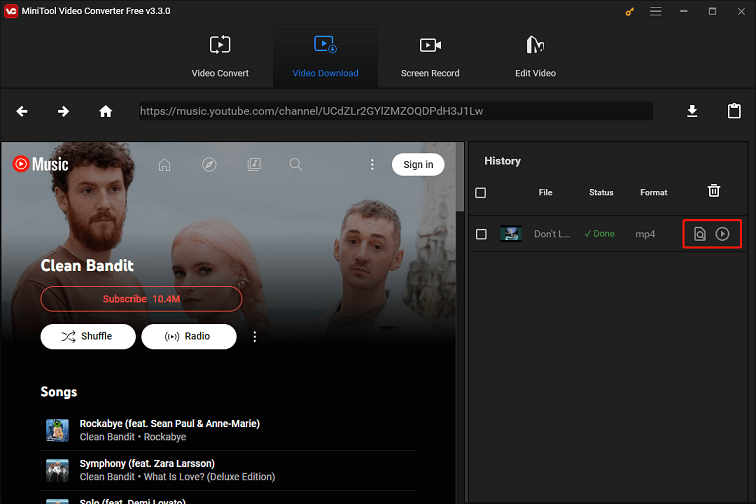The image depicts a web page featuring a video editor for YouTube named MiniTool Video Converter Free V 3.3.0.

In the upper left-hand corner of the web page, there is a small red square with white text inside it that reads "VC." Adjacent to this square, the page title identifies the software as "MiniTool Video Converter Free V 3.3.0."

The upper right-hand corner of the web page displays a series of symbols: a yellow key, a horizontal line, a subtraction sign, a window icon, and an "X" symbol, listed from left to right.

Centered in the middle of the page, there are four categories, each represented by white hollowed-out icons and text. The categories are listed from left to right as "Video Convert," "Video Download," "Screen Record," and "Edit Video." The "Video Download" category is highlighted in blue, distinguishing it from the others.

Below the category menu, a search bar is visible. It contains a link to a music YouTube channel, flanked by a white home symbol and left and right-facing arrows on the left side. On the right side of the search bar, there are icons for downloading and copying to the clipboard, arranged from left to right.

Towards the lower left part of the image, three people are standing against a background, featuring the text "Clean Bandit" in white overlaid on them. The man on the left has red curly hair and a red beard. The person in the middle is shorter and has pink hair. The person on the right has short hair, is staring directly at the camera, and has a faint mustache.

Underneath "Clean Bandit," there is a red subscribe button indicating "10.4 million" subscribers. Below this, there are two white pill-shaped buttons, one for shuffle and one for radio. Further down, several songs are listed alongside partially visible album artwork. The song titles are "Rockabye" featuring Sean Paul and Anne-Marie, "Symphony" featuring Zara Larsson, "Clean Bandit What Is Love," and "Clean Bandit Rockabye."